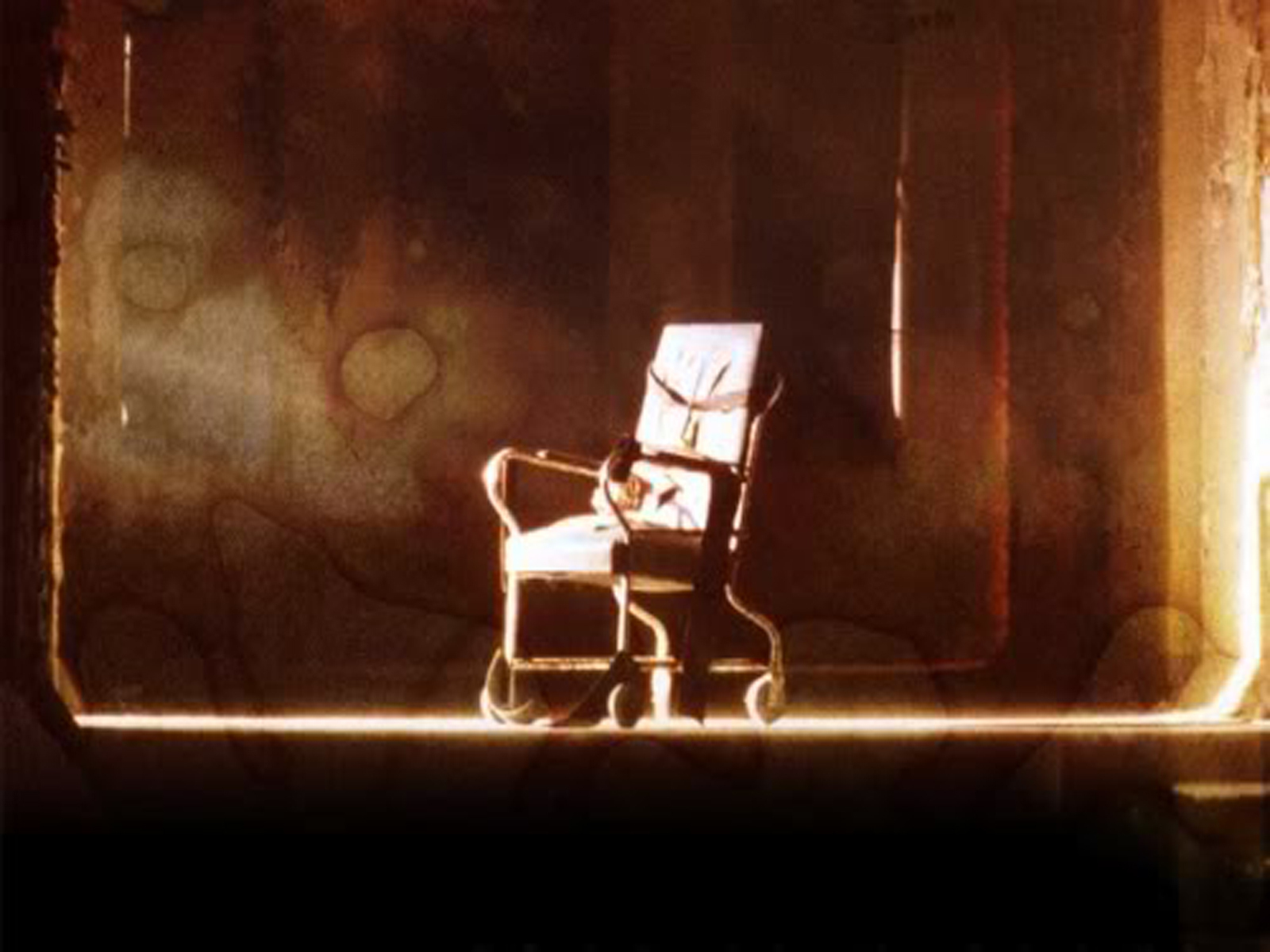This is an antique-looking photograph, likely a still from a horror film, depicting a dilapidated old barn. At the center of the barn's floor is an eerie, vintage wheelchair. The wheelchair resembles those once used in psychiatric wards, with multiple restraining straps designed to secure a patient. There are straps for the upper torso, waist, and legs, as well as additional straps on the armrests to immobilize the person's arms. The scene conveys a chilling and unsettling atmosphere, heightened by the sinister implications of the wheelchair's purpose.